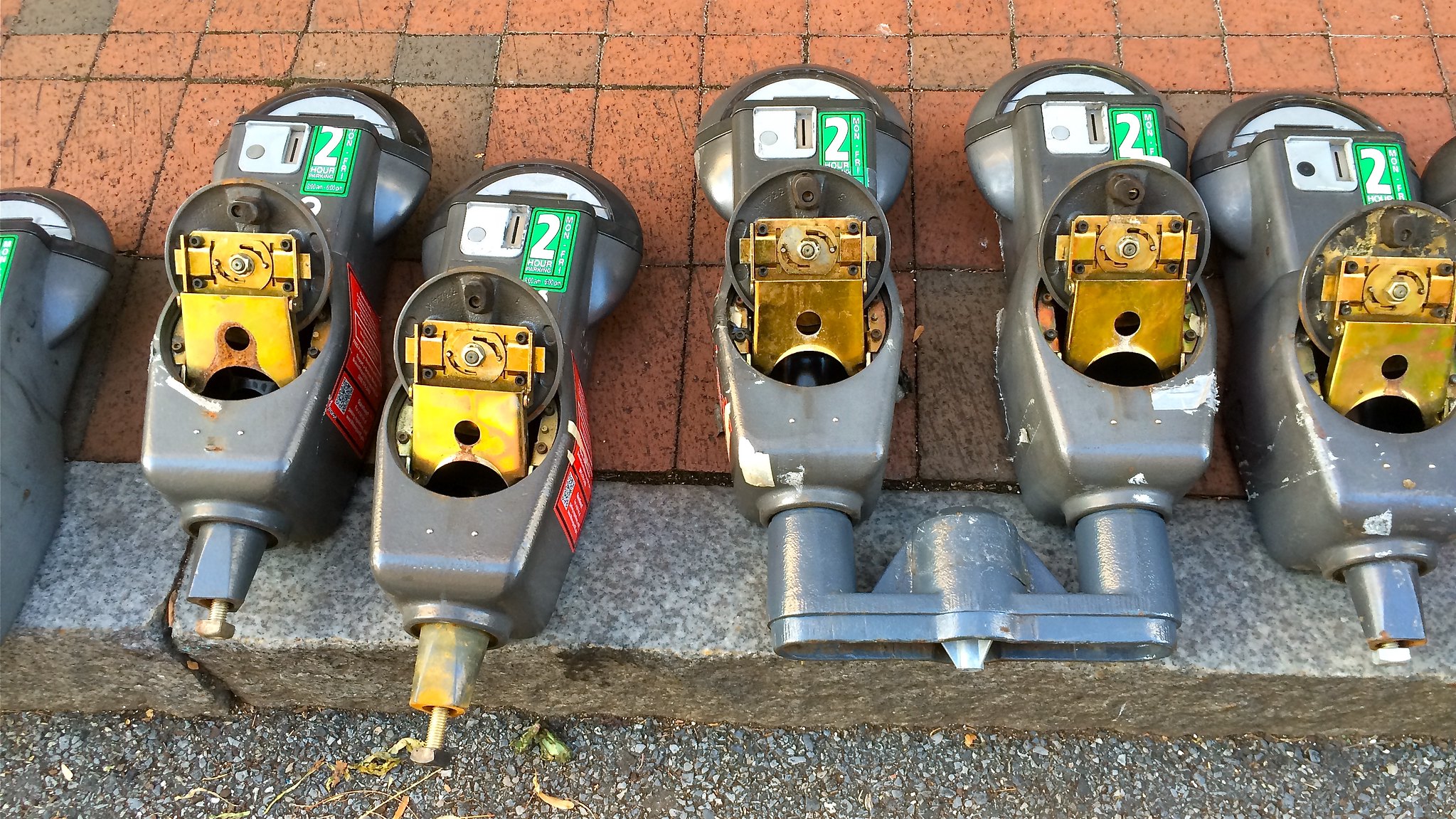This detailed color photograph captures the detached heads of six silvery parking meters laid out on a reddish brick-paved sidewalk, adjacent to a granite curb. Each meter head features a distinctive structure: a yellow center, a white top section, and a green sticker labeled with the number "2" on the right-hand side. The photograph, taken from a 45-degree top-front angle, showcases the internal components of the meters, with some revealing frayed cores and brass elements inside. Among the six, four are single units while one is a dual configuration, joined together for dual installation on a single pole. Visible bolts and nuts on three of the meters indicate where they would attach to their respective poles. The lower edge of the image shows a grey gravel area with a few green leaves scattered about, enhancing the overall scene.